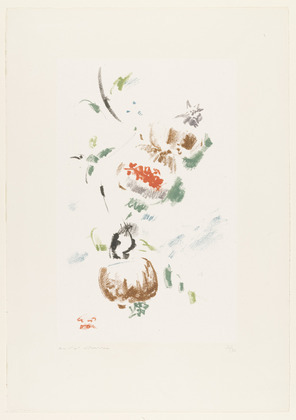The image depicts an abstract painting with an off-white or canvas-white background that is bordered by a faint white outline, resembling either a book cover, postcard, or a traditional painting. At the center of this vertically oriented rectangle, various shapes and brushstrokes converge to form a vague but evocative composition. 

Starting from the bottom, there is a dominant brown circular shape, somewhat resembling a bowl or vase, embellished with hints of white, suggesting a planter of some sort. Beside this brown circle are three horizontal stripes: two shades of green and one gold. Two black lines extend upwards from this region, intertwining with green squiggles that meander into a mixture of gray and red areas, possibly suggesting either leaves, vines, or an abstract representation of fruit.

Above the primary brown shape, several green blotches and streaks span the composition. Two parallel black blotches framed by green emerge towards the middle, intersected by an arc of green transitioning into wider black and red stripes. This culminates in another brown curved form with additional brown shading above. At the very top of the image, there exists a star or flower shape rendered in shades of gray or violet.

The entire scene appears as an abstract portrayal of a plant in a vase, enhanced by varied brushstrokes and splashes of color that invoke organic forms and natural elements without committing to any specific representation.